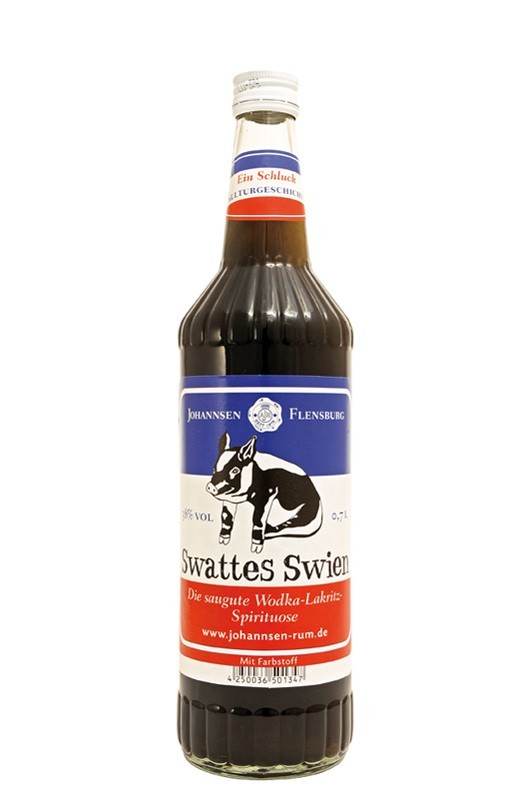The image depicts a single, large bottle centrally positioned against an all-white background, ideal for a product webpage. The bottle appears to be made of either plastic or glass, filled with a dark brown liquid resembling cola or rum. The main label on the bottle features a mix of colors: red, white, blue, brown, and black. Notably, there is a black and white cartoon pig depicted prominently on the label. Text across the label is mostly in German, with key phrases such as "Johansson Flensburg" and "Swatty Swine." Additional details include blue, white, and red stripes on both the main label and a smaller label near the white cap. Further text indicating the website "www.johansson-rum.de" suggests the product may be a spirit, possibly vodka or rum. A barcode is present at the bottom of the label. The overall sharpness and composition, with the bottle perfectly centered, reinforce its use for a professional product listing or advertisement.